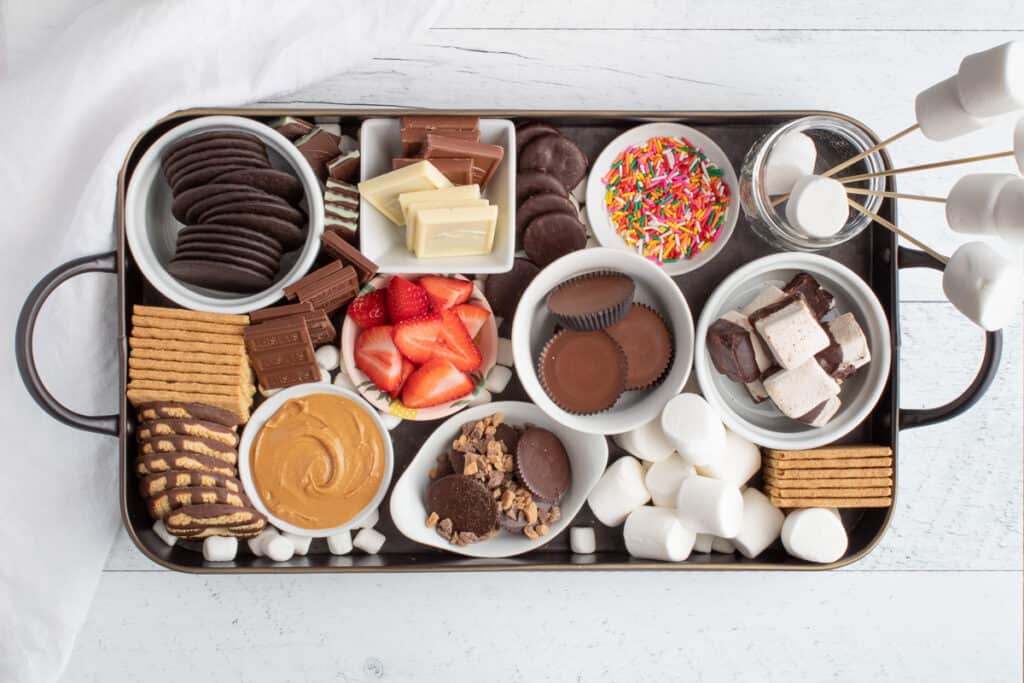This image features a meticulously arranged dessert charcuterie board captured from a top-down perspective. Presented on a dark, almost black metal tray, the assortment includes a variety of sweets packed together, filling the entire tray. Among the treats are numerous small white dishes containing different snacks. Key items include a glass jar in the top right corner, holding marshmallows on sticks with two loose marshmallows inside. Nearby, a bowl of rainbow-colored sprinkles (or jimmies) sits beside six thin mints and a bowl with both white and dark chocolate squares. Six Andes mints and a tray of chocolate-covered cookies anchor the assortment, alongside a variety of graham crackers and other cookies. There are also more marshmallows and graham crackers scattered around, and two bowls filled with Reese's peanut butter cups, one mixed with Reese's pieces. Additional bowls feature items like marshmallow squares, halved strawberries, and plain peanut butter. The entire setup is laid out against a background resembling white-painted wood, with a corner of a white tablecloth visible in the top left. The collection of chocolates, crackers, marshmallows, and other sweets suggests it may be intended for making gourmet s'mores.